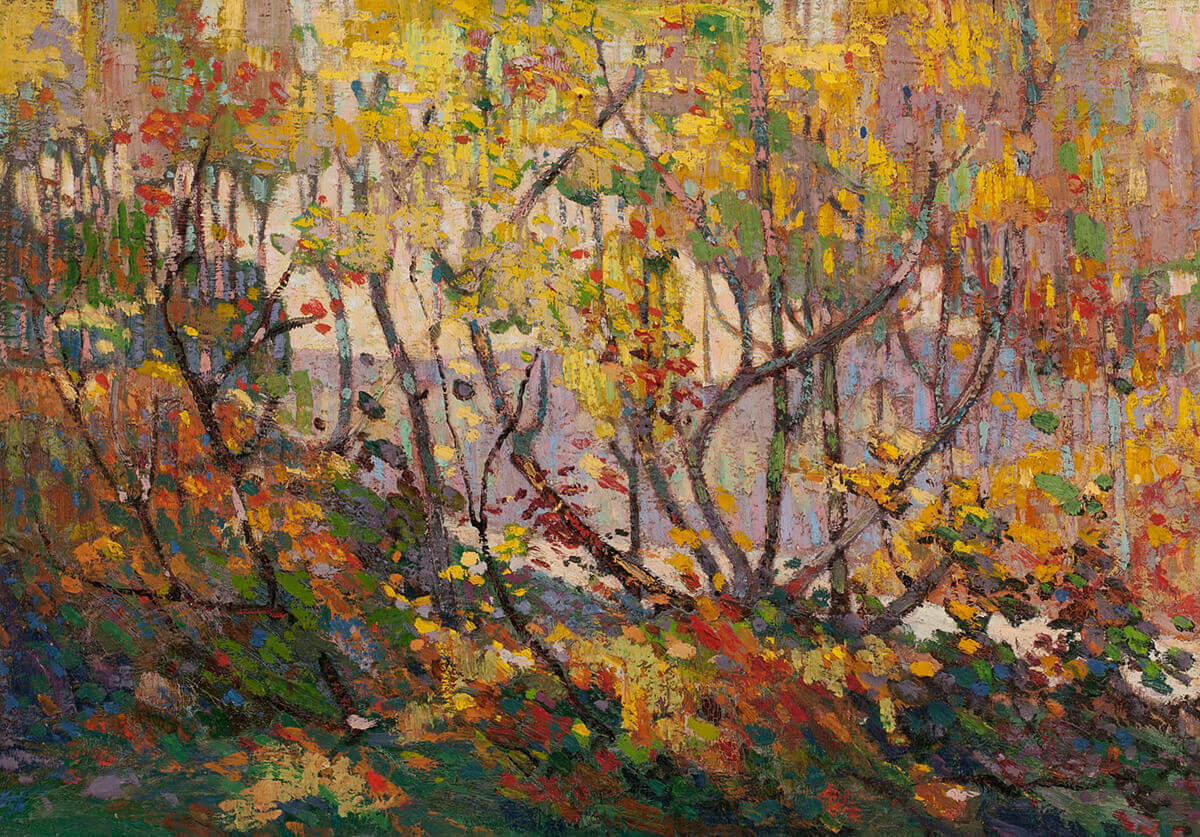This image is a warm, vivid impressionist painting, likely created in a pointillism or dotwork style. The painting is rich in colors, including green, orange, gray, black, red, yellow, blue, purple, pink, and tan. The scene features a vibrant depiction of nature, with a large grassy area at the bottom of the image transitioning into a forest floor. From this grassy area, trees with thin branches and leaves in vivid greens and yellows, along with some red and gray, rise towards the top of the image. The tree trunks and branches, painted in brown or dark gray, swirl elegantly upwards. There's a body of water positioned near the center of the image, behind the trees, rendered in bluish and pinkish hues with patches of color that resemble reflections of the trees. The water extends up to the middle part of the painting, possibly hinting at a beach area in the upper section. The overall composition of the painting is abstract yet detailed, with no text visible, making it a piece one might expect to see hanging in someone's home.